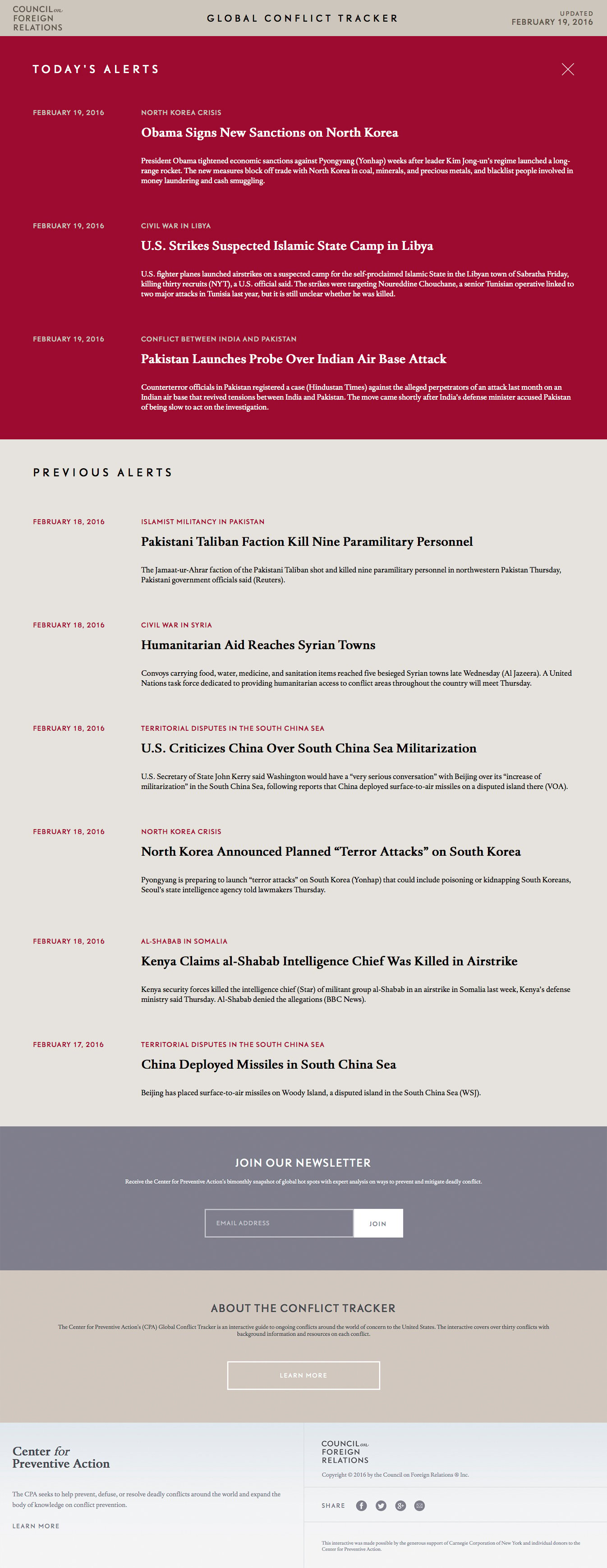The image appears to be a low-quality snippet from a newsletter focused on geopolitical alerts. Despite its small size, several distinct sections and textual elements are discernible.

At the top of the image, a beige strip contains the title "Global Conflict Tracker" in prominent black capital letters. Adjacent to this title on the left side, there is what seems to be a logo, comprising three lines of black text, the specifics of which are indiscernible due to low image quality.

Below this, the newsletter features a rectangular section with a deep royal red background. On the left side of this red area, there is white text with significant letter-spacing that reads "TODAY'S ALERT." 

Underneath the "TODAY'S ALERT" title, three sections are spaced out toward the right with bold white headlines. These include:
1. "Obama signs new sanctions on North Korea."
2. "US strikes suspected Islamic State camp in Libya."
3. "Pakistan launches probe over India air base attack."

Following this, the lower half of the image is dominated by a larger beige section, approximately double the size of the red area above. In the upper left corner of this beige section, the text "PREVIOUS ALERTS" is displayed in black capital letters. Several bold headlines are listed below this heading:
1. "Pakistan: Taliban faction kill nine preliminary personnel."
2. "Humanitarian aid reaches Syrian town."
3. "US criticizes China over South China Sea militarization."
4. "North Korea announces planned terror attacks on South Korea."
5. "Kenya claims Al Shabaab intelligence chief was killed in airstrike."
6. "China deployed missiles in South China Sea."

Due to the low image quality, this detailed description may contain minor inaccuracies regarding specific text.